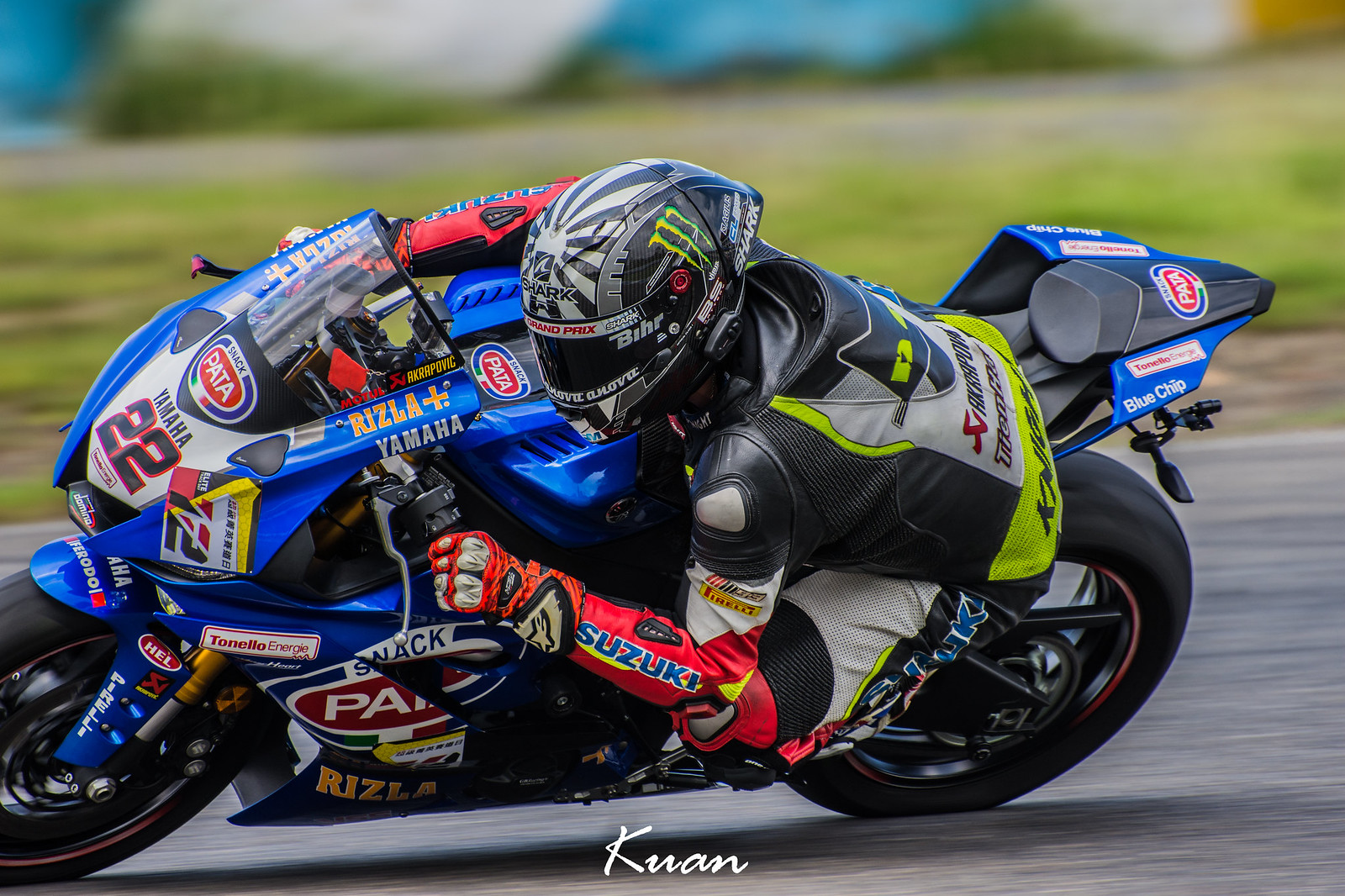This is a horizontally oriented photograph capturing a motorcycle racer, whose gender is indeterminate due to a helmet, protective gloves, and a uniform. The shot, a side profile, shows the rider and their blue Yamaha motorcycle leaning sharply into a turn, with the vehicle's front oriented to the left and rear to the right. The motorcycle is adorned with various colorful advertising stickers, including prominent ones from Yamaha, Monster Energy Drink, and Suzuki, as well as blue chip PATa and ARIZLA. The rider's black helmet also features white graphics and advertising logos. Their racing suit is predominantly black, yellow, and white, with flashes of orange on the gloves and knee pads. The motorcycle is fitted with large tires, accentuating its racing design. The background features a blur of green grass and road, underscoring the high speed at which the racer is moving, while the focus remains crisp on the motorcycle and rider. A watermark with the letters "KUAN" is visible at the bottom center of the image.